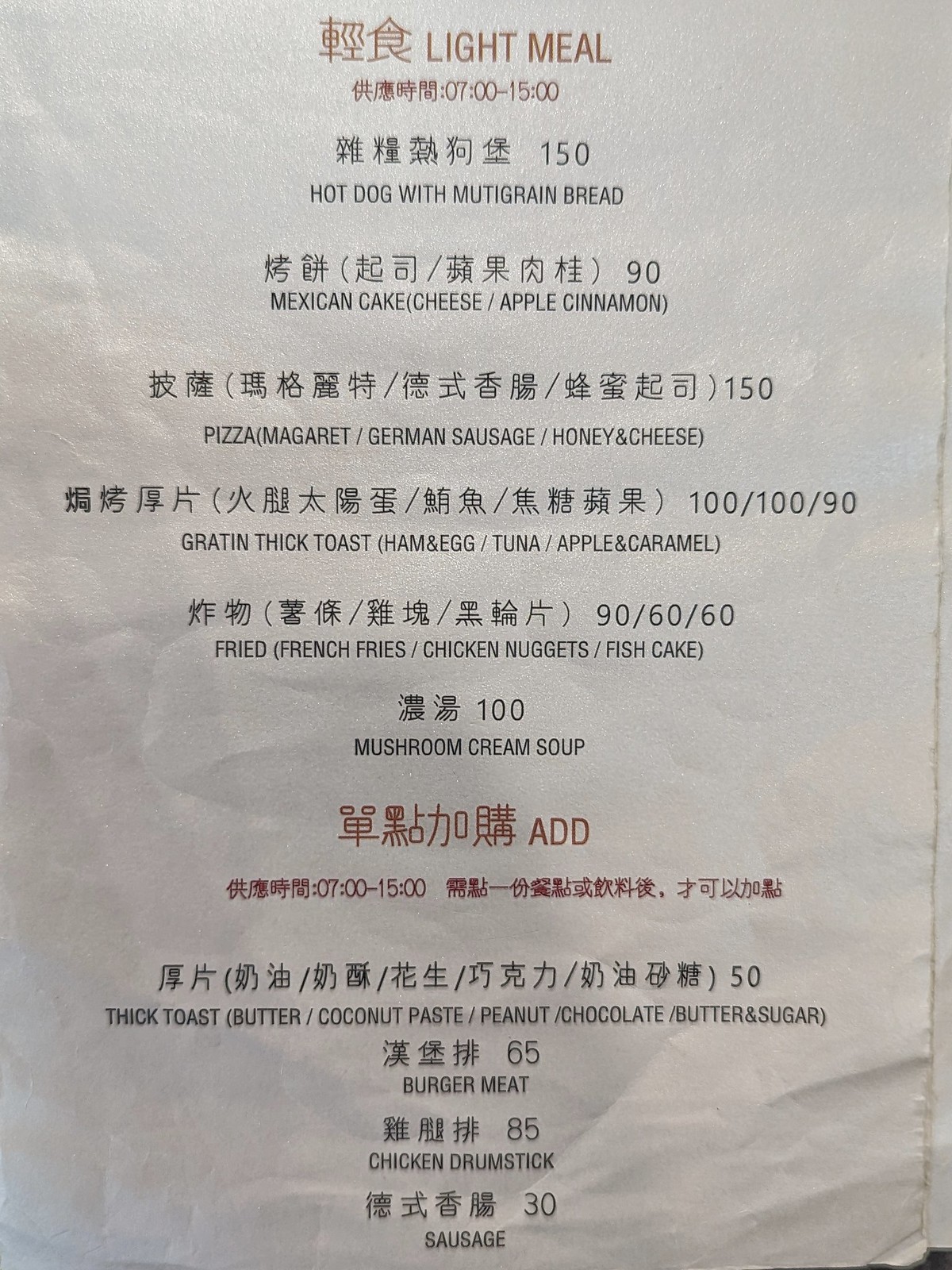The image depicts a wrinkled white piece of paper, serving as a menu, with both English and Chinese text, featuring black and red letters. The menu lists various items with corresponding prices, likely in yen, each accompanied by Chinese symbols providing translations. At the top, the menu offers a "Hot Dog with Multigrain Bread," followed by a "Mexican Cake / Cheese" and "Apple Cinnamon," priced at 90 yen.

Other items include:
- "Pizza Margaret / German Sausage / Honey and Cheese"
- "Garlic Thick Toast / Ham and Egg / Tuna / Apple and Caramel" for 100 yen or 90 yen
- "Fried French Fries, Chicken Nuggets, and Fish Cake" priced at 90 yen, 60 yen, or 60 yen respectively
- "Mushroom Cream Soup" for 100 yen
- "Thick Toast with Butter, Coconut Paste, Peanut, Coconut Butter, and Sugar" for 50 yen
- "Burger Meat" for 65 yen
- "Chicken Drumstick" for 85 yen
- "Sausage" for 30 yen

This menu, with its mix of languages and detailed dish descriptions, appears to be reflective of an Asian restaurant's offerings, providing a diverse selection of foods along with their prices.